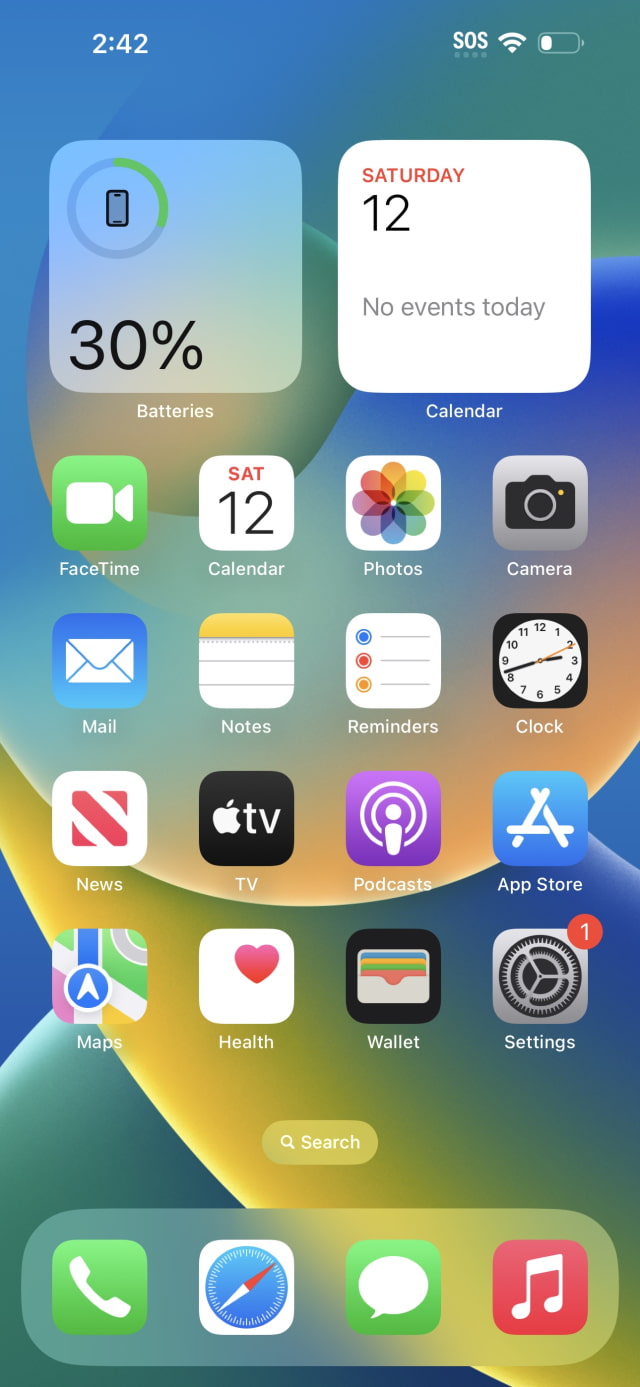This image showcases the home screen of an Apple iOS device. In the top left corner, the battery icon indicates a 30% charge remaining. Adjacent to this, a calendar widget displays "Saturday 12th" with a note stating "No events today", set against a white background.

The home screen features a 4x4 grid of 16 app icons, with an additional 4 app icons docked at the bottom, totaling 20 apps. The background of the screen is a vibrant gradient comprising shades of yellow, blue, and hints of green.

The docked apps at the bottom, listed from left to right, include:
1. Phone (green and white)
2. Safari browser (blue and white with some red)
3. Messages (green and white)
4. Apple Music (red and white)

The 16 apps displayed in the grid, starting from the top left, are:
1. FaceTime (green and white)
2. Calendar (white, black, and red)
3. Photos
4. Camera
5. Mail (blue and white)
6. Notes (white and yellow)
7. Reminders
8. Clock (black and white)
9. News
10. Apple TV (black and white)
11. Podcasts (purple and white)
12. App Store (blue and white)
13. Maps
14. Health (white and red)
15. Wallet
16. Settings (which has one notification badge)

Each app icon is clearly illustrated, contributing to a well-organized and visually pleasing home screen.